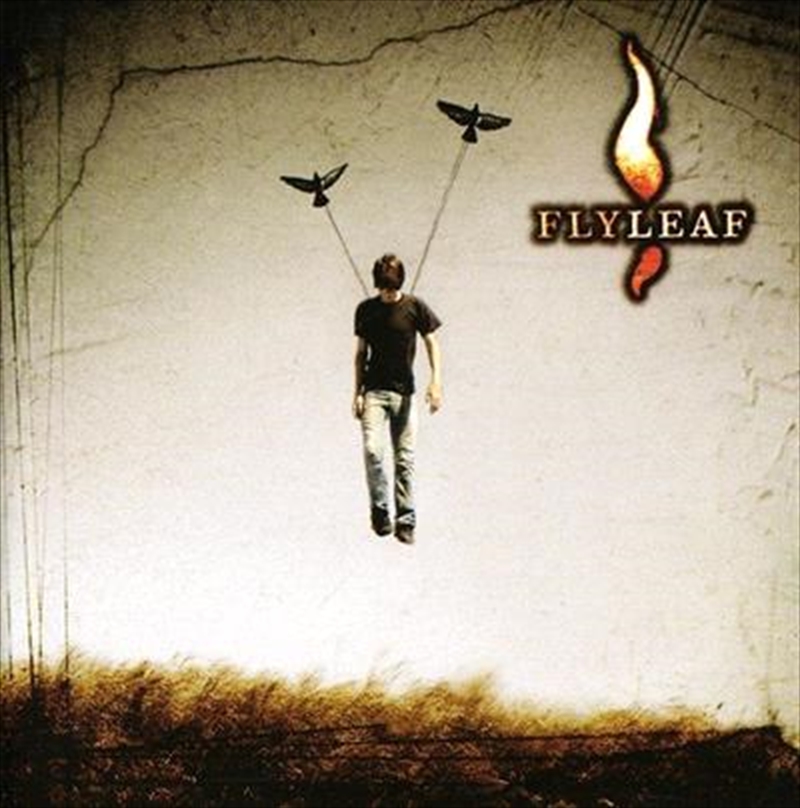This color image appears to be an artistic album cover, likely for the band Flyleaf, as their name prominently appears in the upper right corner, with distinctive flames shooting both up and down between the "L" and "E" in "Leaf". The background is predominantly white, featuring black cracks that add a dramatic effect. At the center of the image, a human male dressed in a t-shirt and blue jeans is depicted floating mid-air in a pose that suggests he is walking. Interestingly, he is tethered to two black birds by strings attached to his shoulders, giving the impression that the birds are lifting him. Below this dynamic scene, a field of brown, hay-like grass completes the setting.